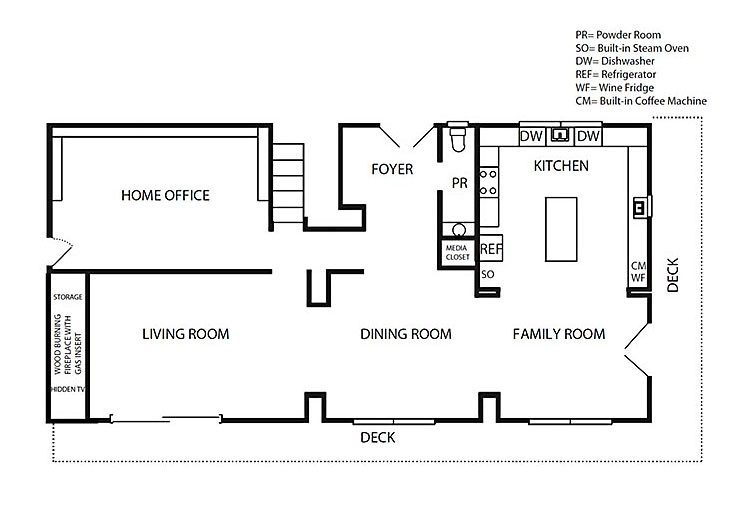The image features a detailed floor plan of a house set against a plain white background. The floor plan is rendered in black text and lines, resembling a professional architectural drawing viewed from above. 

The house is a horizontally oriented rectangle. Notable rooms and features are labeled as follows:

- **Top Left:** Home Office
- **Top Middle:** Foyer
- **Top Right:** PR (Powder Room)
- **Underneath the Powder Room:** Media Closet
- **Right of Media Closet:** Kitchen

In the kitchen:
- **Top:** Two "DW" signs indicating the Dishwashers
- **Left:** "REF" denoting the Refrigerator
- **Bottom Left:** "SO," for the Built-in Steam Oven
- **Right:** "CM," indicating the Built-in Coffee Machine
- **Bottom Right:** "WF," signifying the Wine Fridge

In the bottom left corner:
- Storage
- Hidden TV
- Wood-Burning Fireplace with Gas Insert

Other main areas:
- **Bottom Left:** Living Room
- **Bottom Middle:** Dining Room
- **Bottom Right:** Family Room

An L-shaped deck runs around the lower right side of the house. The top right corner of the plan includes a legend clarifying the shorthand letters used in the labeling.

Overall, this floor plan provides a thorough and comprehensible layout of the house's interior and designated features.